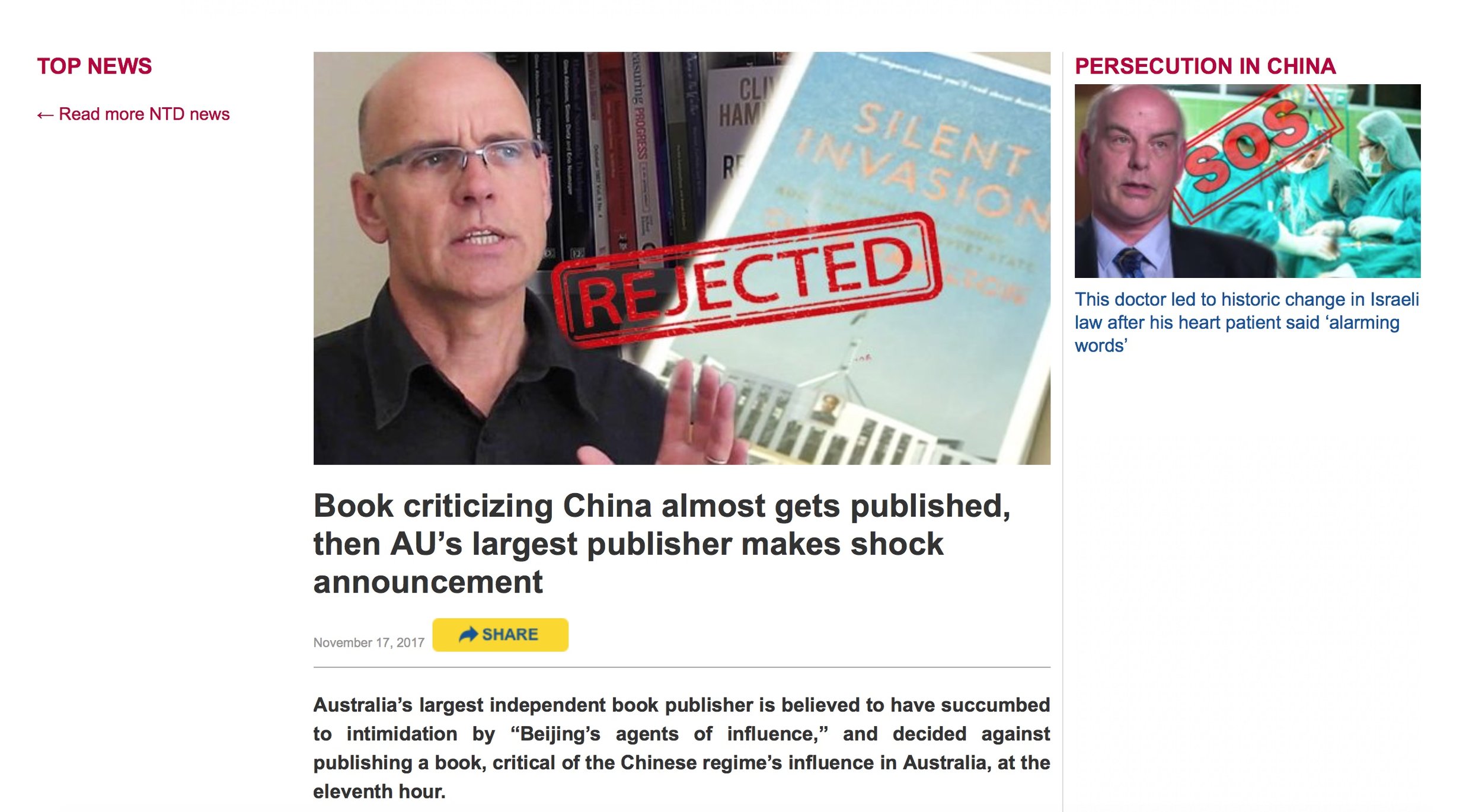The image depicts a section from a news website, specifically under the "Top News" category, highlighted in a purplish font. A left-pointing arrow marked "Read More" and the logo "NTD News" are situated under this heading. The section showcases two articles, each accompanied by an image of a bald white male with distinct red stamps emblazoned on them.

On the left, the first article features a bespectacled white male wearing a black, open V-neck shirt with a collar. The image includes the red stamp "Rejected" overlaid on a book titled "Silent Invasion." Below the image, the headline reads, "Book Criticizing China Almost Gets Published," followed by, "AU's largest publisher makes a shock announcement." A share button is positioned beneath this caption.

To the right, the second article shows another white male, with what appears to be doctors in the background. This image bears a red stamp marked with "SOS" enclosed in a red box border. The headline for this article is "Persecution in China." Below both headings, there is additional information formatted into a paragraph and highlighted in black, though the content is not fully visible in the provided description.